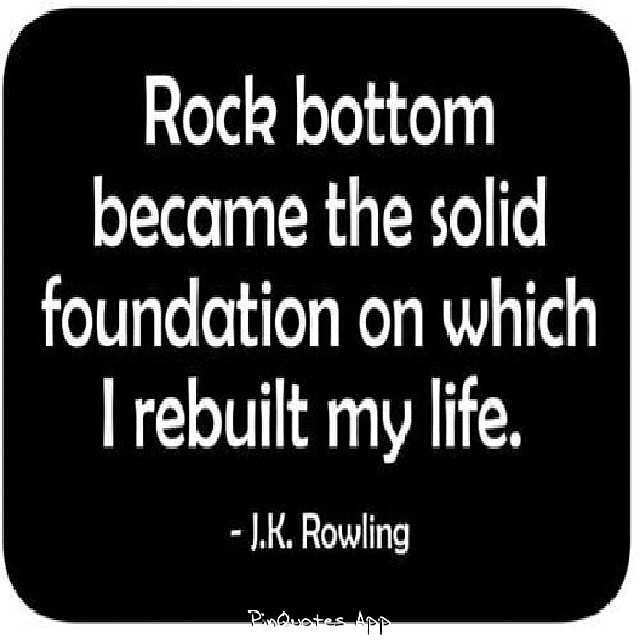The image features a quote by J.K. Rowling, saying, "Rock bottom became the solid foundation on which I rebuilt my life." The text is in a bright, white sans-serif font, making it stand out against the solid black background. The font is bold and neat, with the words "rock bottom became the solid foundation on which I rebuilt my life" being the most prominent, while "J.K. Rowling" is presented in a smaller font size below. At the very bottom, in a scratchy handwriting style, it says "Pin Quotes App," though the logo appears slightly cut off. The overall composition of the image is centered, presenting the quote in a clear and impactful manner. The black background has slightly curved edges, adding a subtle touch to the otherwise stark design.